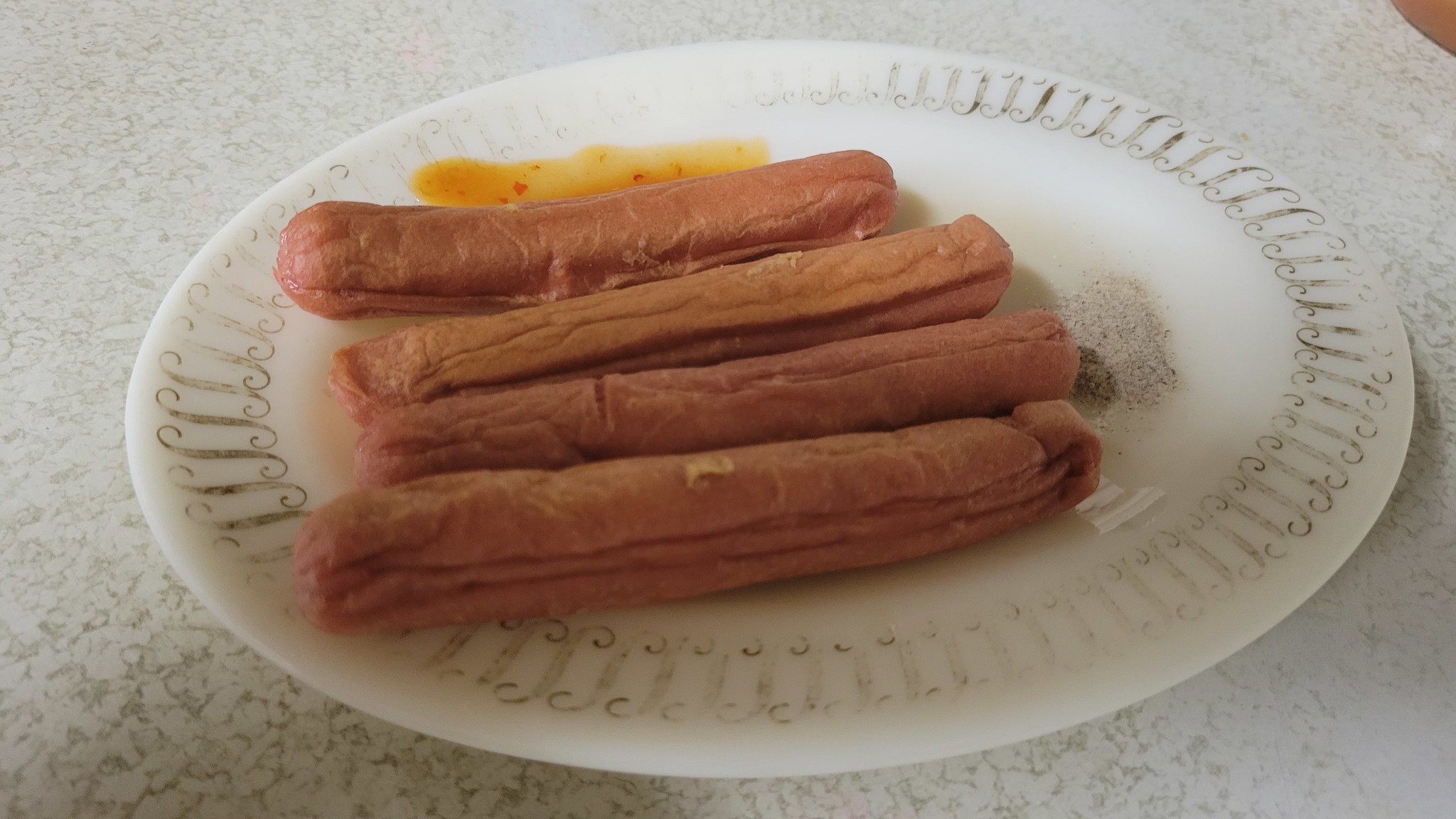This horizontally rectangular photo showcases a white ceramic plate adorned with a detailed brown and silver swirl pattern along the edge. Positioned on the plate are four naked hot dogs, severely overcooked to the point of extreme dehydration, exhibiting pronounced wrinkles and a light brown hue. These hot dogs are surrounded by a hint of what appears to be sauce or perhaps mustard near the top of the frame, and possibly a small pile of pepper or some condiment behind them. The plate itself rests on a formica or granite countertop with a white marble design, contributing an additional textured layer to the background. Overall, the image captures the unappetizing appearance of the shriveled hot dogs in stark detail.